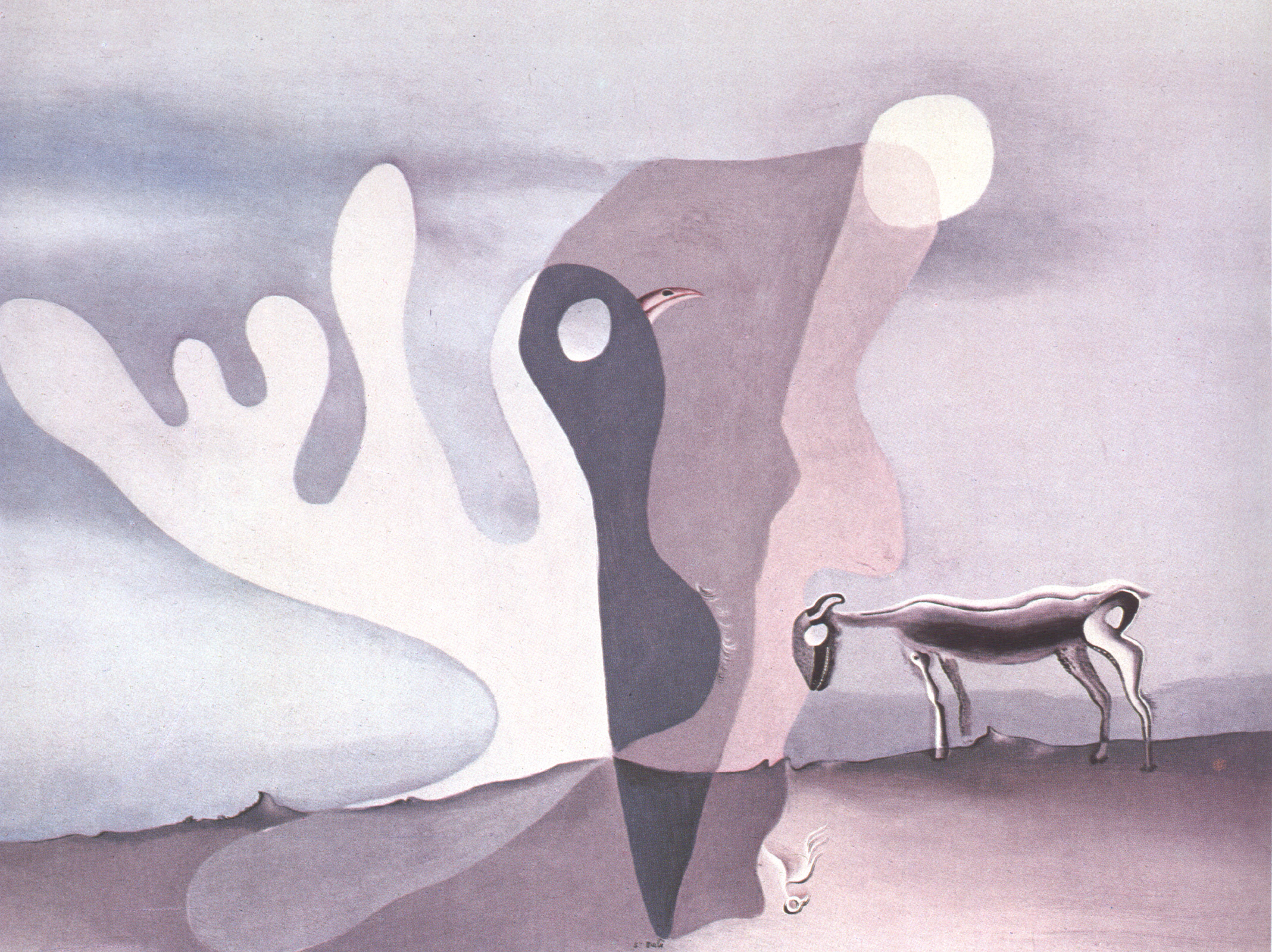This abstract piece of art portrays an outdoor night scene, possibly created with watercolor paints. Dominating the foreground is a large, black-and-white bird with a distinctive beak and a prominent white circle for its eye. The bird is facing to the right and occupies much of the center of the composition. To the right, there is a sketched, possibly hand-drawn, animal that resembles a goat, standing on the ground and facing left. All four legs and a tail are visible. The background features a sky that appears cloudy, with a moon partially obscured by clouds. The predominant colors in this piece are white, black, gray, tan, and brown, contributing to its abstract and somewhat surreal quality. The overall impression is that of a nocturnal scene filled with interesting and ambiguous details, reminiscent of a cartoon or a hand-drawn sketch.